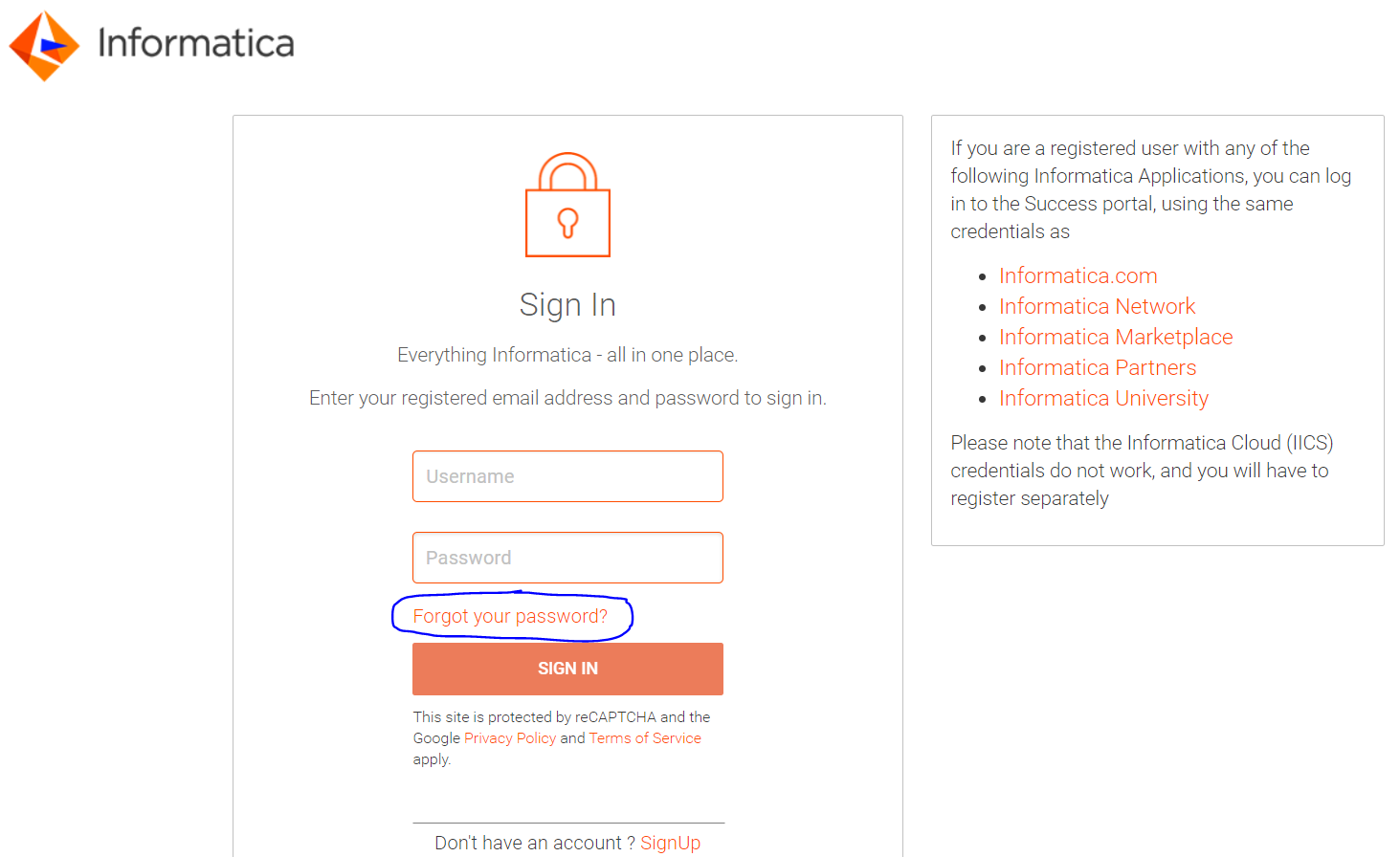This image depicts the sign-in page of the Informatica website, characterized by its distinctive orange diamond-shaped logo that resembles origami. The page prominently features an orange lock icon above the "Sign In" header, followed by the phrase "Everything Informatica all in one place." 

Users are prompted to enter their registered email and password within two input fields, both bordered with an orange outline. Below these fields, there is a "Forgot your password?" option highlighted in orange and circled, drawing attention to recovery options.

An all-orange button with white text labeled "Sign In" is situated beneath the input boxes. Further down, the page notes that "This site is protected by reCAPTCHA and the Google Privacy Policy and Terms of Service apply." 

At the bottom, prospective users are given an option to "Sign up" if they don't have an existing account. 

To the right of the main sign-in area is a secondary box detailing that registered users of any listed Informatica applications, such as Informatica.com, Informatica Network, Informatica Marketplace, Informatica Partners, and Informatica University, can log into the Success Portal with the same credentials. However, it specifically mentions that Informatica Cloud IICS credentials are not applicable, requiring a separate registration.

The layout is divided into two sections: a larger section for the sign-in process and a smaller adjacent box with information for registered users.